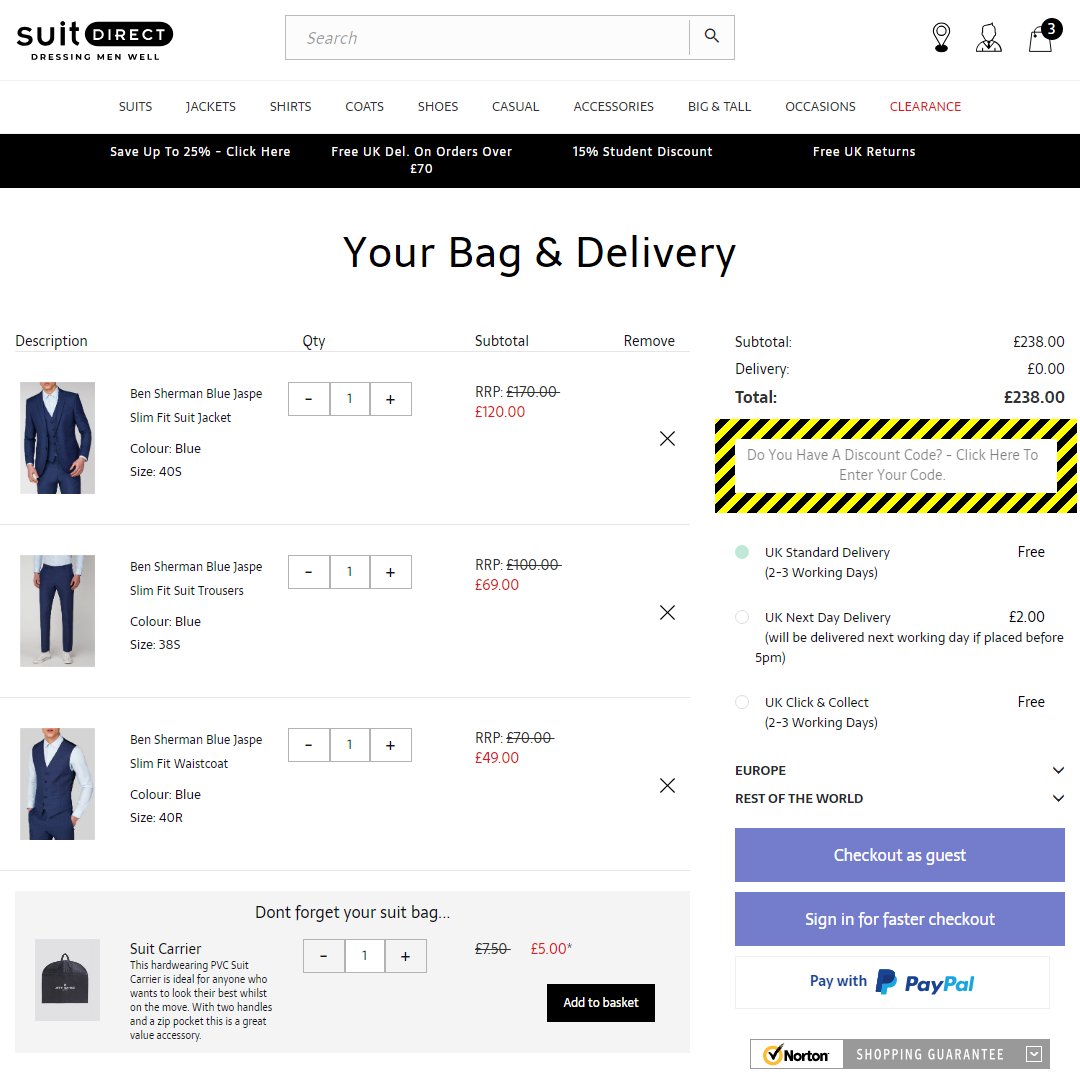This screenshot captures the homepage of a men’s clothing retail website called "Suit Direct." The website’s logo is displayed prominently on the top left, featuring the word "Suit" in bold black text and "Direct" in thin white text within a black, horizontally-oriented oval background. Beneath the logo, the slogan "Dressing men well" emphasizes the site’s focus on men’s formal wear.

Centered at the top is a rectangular search bar, facilitating easy navigation. On the top right, there are icons for user-oriented features: a location marker for determining shipping costs and currency, a user profile icon, and a shopping bag symbol with a black numeral "3" indicating the number of items currently in the cart.

Visible at the bottom of the screenshot are three products, presumably the items in the shopping cart. The first item is a Ben Sherman blue jasp slim-fit suit jacket. The second product listed is a matching Ben Sherman blue jasp slim-fit suit trousers. Lastly, a Ben Sherman blue jasp slim-fit waistcoat completes the trio, suggesting a coordinated three-piece suit ensemble.